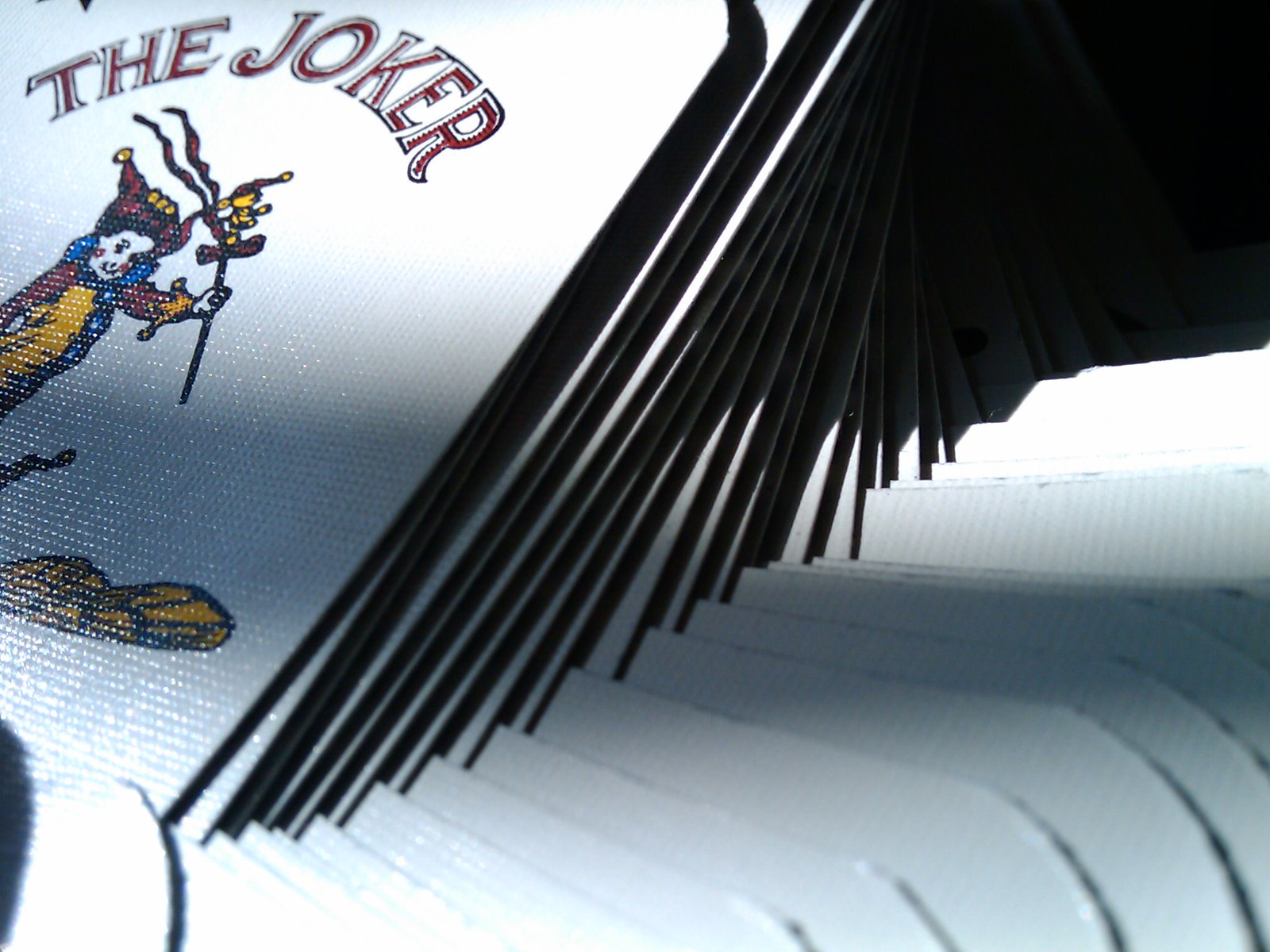The image depicts a surreal, optical illusion scene where stacks of thick poster board or cardboard, possibly wall posters, are arranged in a seemingly chaotic manner. They are splayed out in various directions, creating an effect where it's difficult to determine if they are jutting out of the ground or extending towards the ceiling or walls.

In the center of the viewable stack, one poster is clearly visible, showcasing an illustration of a clown, either a child or a man, holding a staff adorned with ribbons. Above this clown, the word "Joker" is prominently displayed in a font reminiscent of playing cards. The clown appears to be standing over an ambiguous yellow object which could be interpreted as rocks, an animal, or even a body. The entire scene is both intriguing and unsettling, reminiscent of an abstract art piece or a complex visual puzzle.